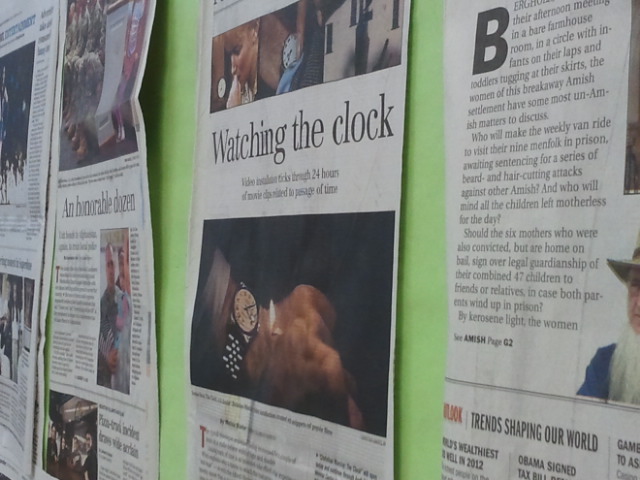This is a square-cropped photograph of a lime green wall adorned with various entire pages from newspapers, captured from a steep angle with the right side of the image closer than the left. Four main newspaper articles are prominently displayed. The central article, "Watching the Clock," features several images including a woman's wristwatch, an up-close shot of a watch face, a wrist with a wristwatch, and a lit match held up to a watch to read the time. Another article on the left is partially readable, titled "An Honorable Dozen," with a visible picture below it. The rightmost article seems to feature an image of an old Amish man, with the text "See Amish Page 2" at the bottom. The print beneath the "Watching the Clock" headline is blurry and unreadable, and while the other two newspapers include pictures, their content is obscured due to the angled perspective.